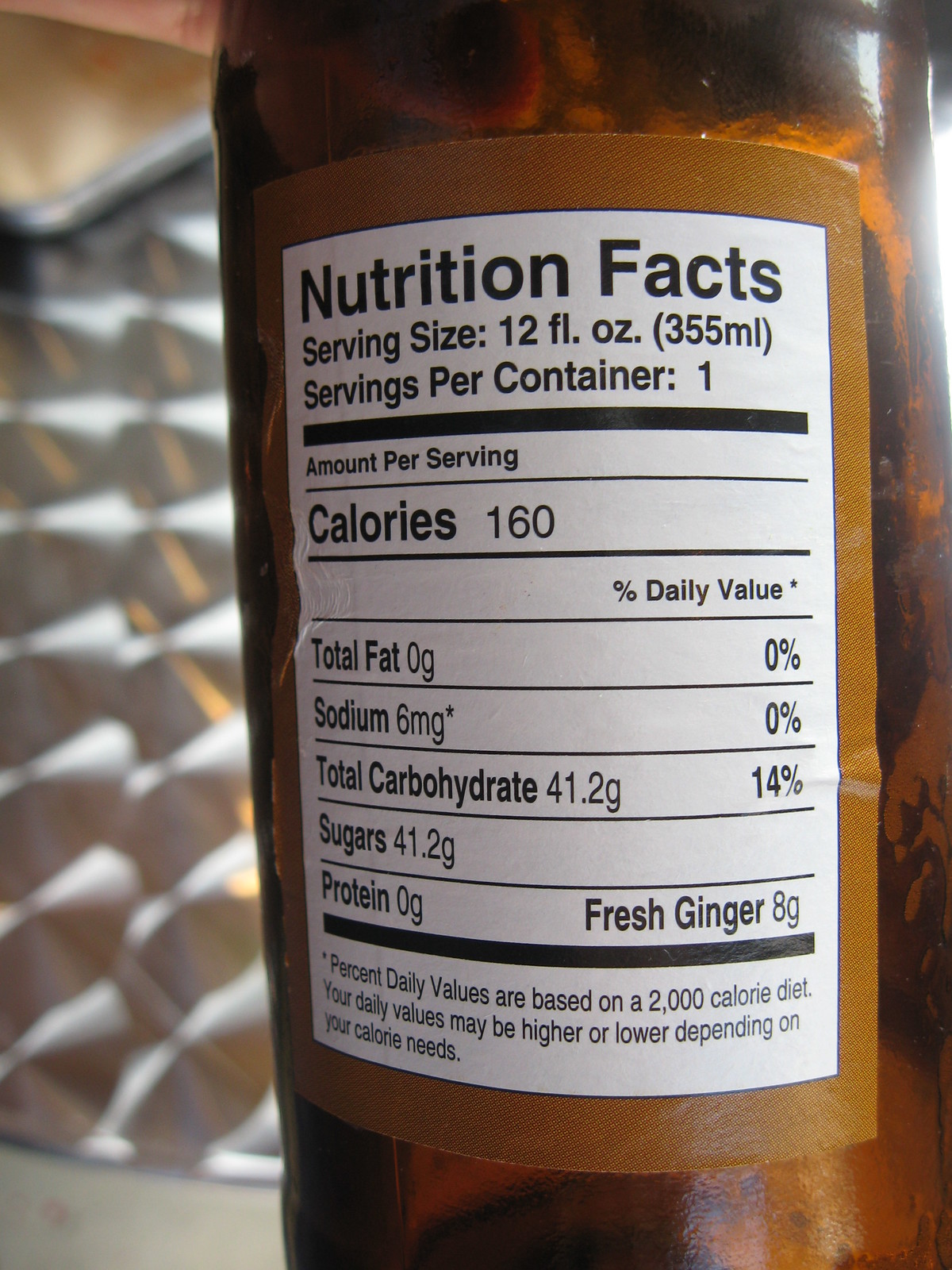This image showcases a glass bottle filled with an amber liquid, prominently displaying a detailed nutritional label. The bottle is set against a backdrop featuring a shiny, chrome-like surface. The label itself is highlighted with a brown outline and a crisp white background, clearly stating "Nutrition Facts." The serving size is specified as 12 ounces, with the entire bottle constituting one serving. Key nutritional information includes 8 grams of fresh ginger, 160 calories, 0 grams of fat, 6 milligrams of sodium, 41.2 grams of carbohydrates (all from sugars), and 0 grams of protein. The label also notes that the percent daily values are based on a 2,000 calorie diet, with individual caloric needs potentially varying.